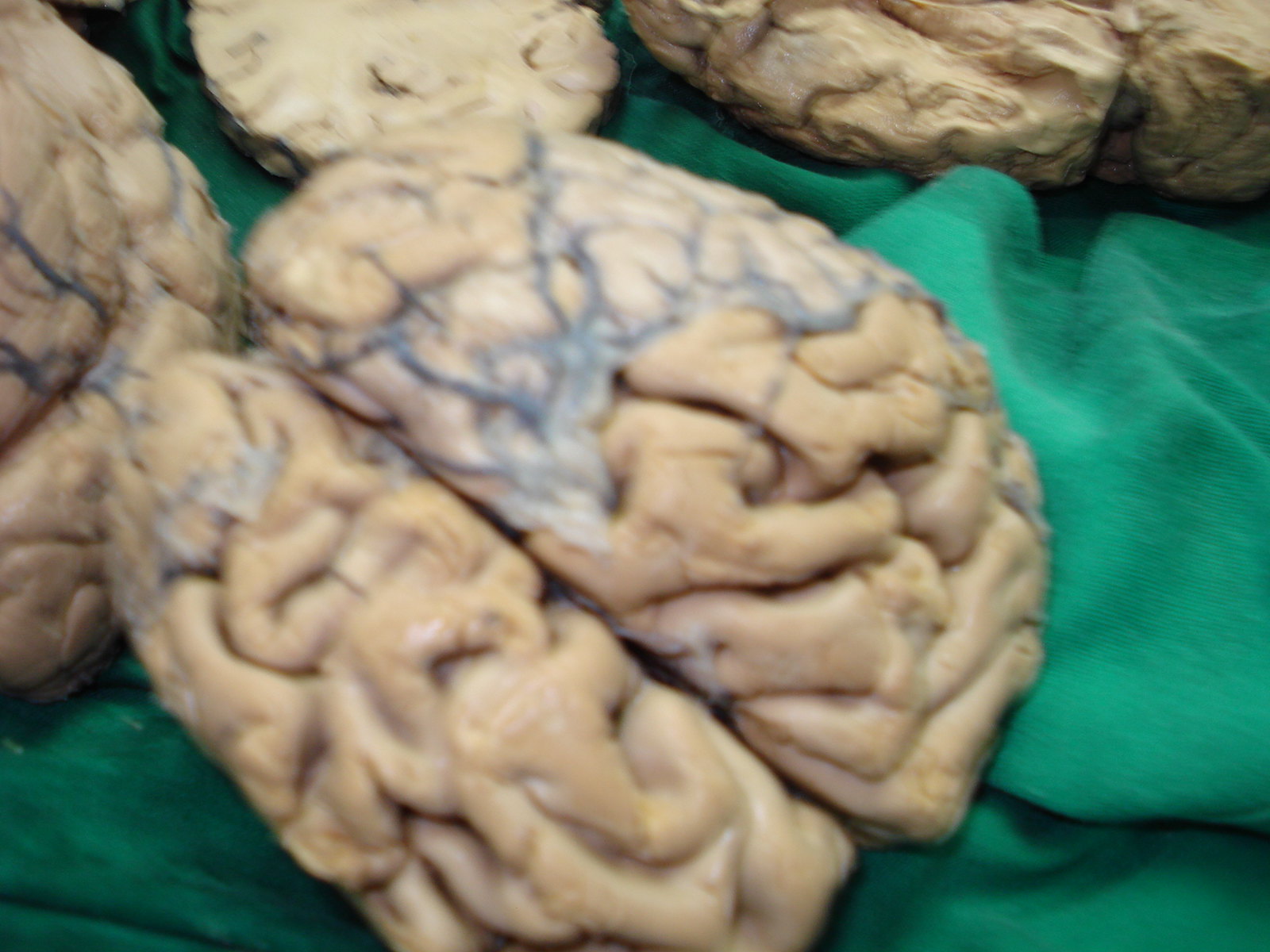This striking and somewhat disturbing image displays several realistic brain-like objects arranged on a bunched-up, thick light green cloth, almost appearing as if they are part of a medical display or possibly very high-quality props. The brains are extremely lifelike with intricate details, including the characteristic two lobes, extensive wrinkles, and dark veins that lend them an authentically flesh-colored, veiny appearance. One brain, prominently positioned in the bottom left, is notably larger than the others, while at the upper part of the image, there's a clear cross-section of a brain, showcasing its internal structure. The brains vary in size and positioning, with some partially obscured or overlapping, adding to the chaotic and jarring scene. The brains rest on a turquoise green material that is not flat but gathered in folds and creases, enhancing the surreal and unsettling atmosphere of the image.